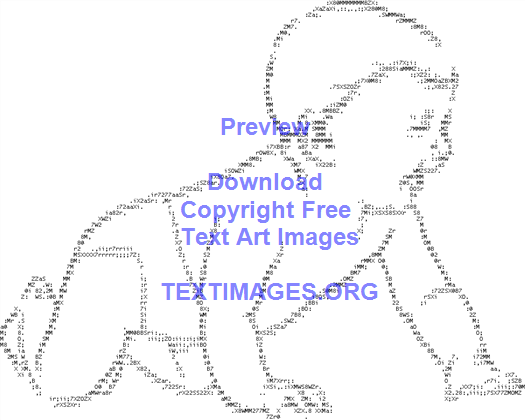The image showcases a piece of ASCII art depicting a baby crawling to the right, primarily crafted using an array of keyboard characters, numbers, and letters. The baby, smiling and wearing a diaper, is intricately outlined and shaded in black text against a stark white background, evoking the appearance of an old dot matrix printout. Superimposed in the center of the image is a line of blue text that reads, "Preview, Download Copyright Free Text Images, textimages.org," indicating that this artwork is part of a collection available for download on that website.